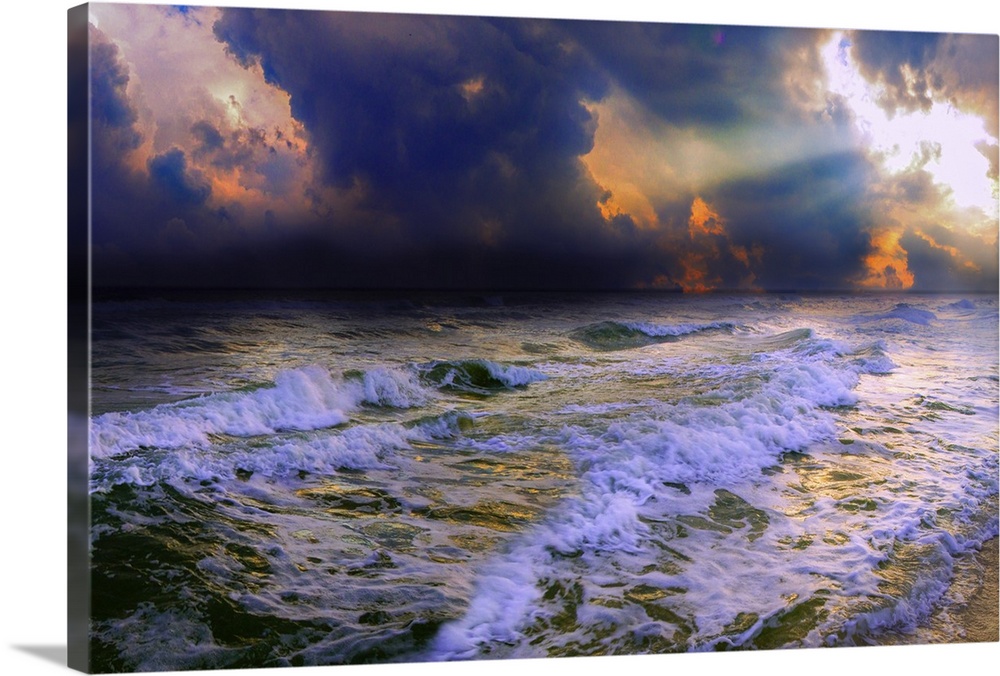This product photograph features a canvas print showcasing a dramatic ocean scene. The professionally edited image places the canvas against a seamless white background, emphasizing the product for online shops, websites, and catalogs. The canvas print depicts a turbulent green ocean with white-capped waves crashing towards a beach in the bottom right corner. The water transitions from green to dark blue as it stretches towards the horizon. Above the restless sea, a sky filled with dark gray clouds looms, with a break in the clouds allowing rays of sunlight to shine through, creating a radiant effect from right to left. Some parts of the sky feature a striking contrast, transitioning from a dark navy blue to a brilliant, blinding white, with hints of golden orange. The photograph of the canvas is angled to reveal its thickness and a soft shadow on the right side, highlighting its three-dimensional quality and adding a sense of depth to the image.